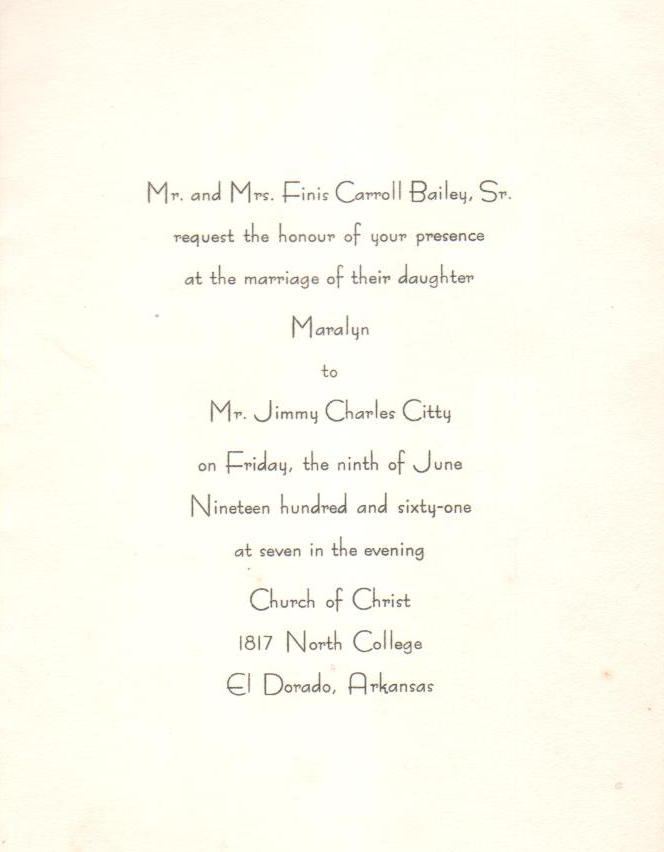This elegantly designed wedding invitation is off-white, resembling a subtle ivory tone. In a simple yet sophisticated black font, it reads: "Mr. and Mrs. Phineas Carroll Bailey Sr. request the honor of your presence at the marriage of their daughter, Mary Lynn, to Mr. G.V. Charles Citty on Friday, the 9th of June, 1961, at 7 in the evening. Church of Christ, 1817 North College, El Dorado, Arkansas." The text is centered, leaving generous space along the top and bottom, accentuating its refined and minimalist design.